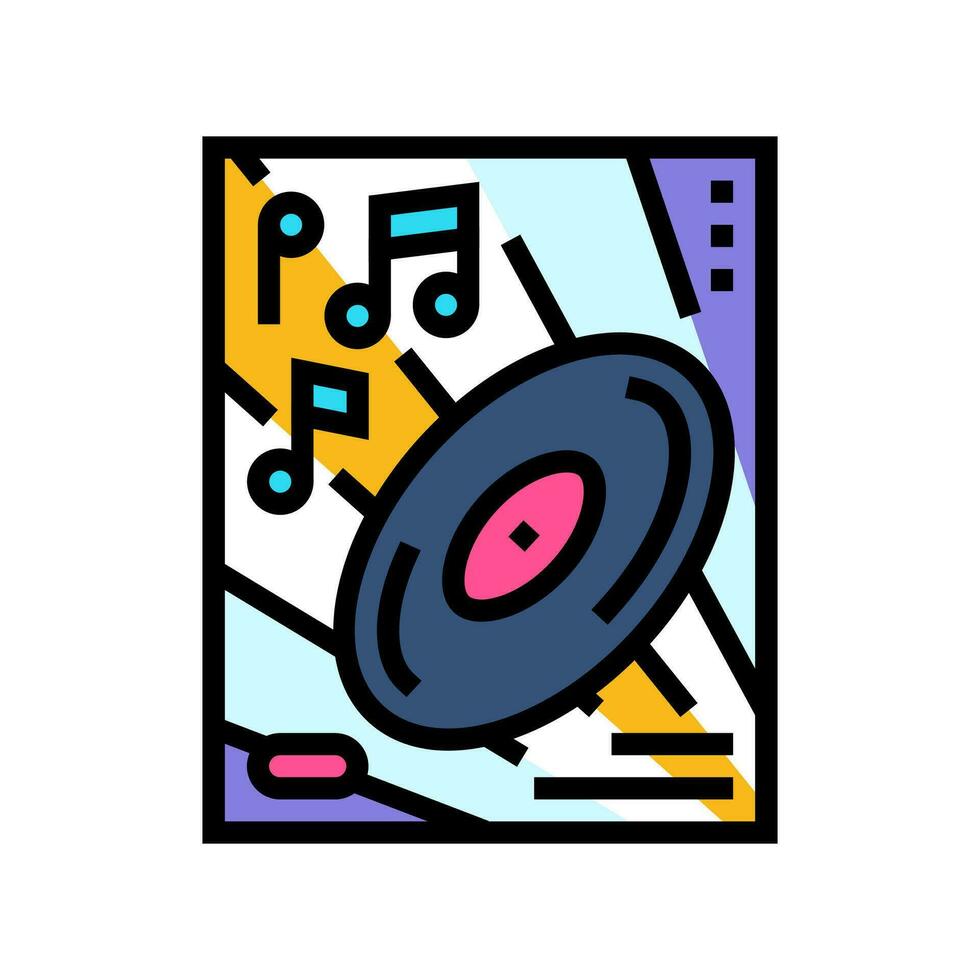This vibrant, digital artwork blends elements of pop art and comic book style to create a nostalgic, music-themed piece. At the center is a diagonal gray record with a pink label, outlined by a black border, suggesting an old-style vinyl. Above and to the right of the record, blue music notes outlined in black visually cue the presence of sound. The background features a dynamic mix of colors: starting from the bottom left corner and stretching diagonally to the top right, there are stripes of purple, light blue, white, yellow, white again, light blue, and another purple box in the top right corner, each stripe outlined in black. The entire composition is framed by a thick black border, enhancing its bold and colorful 50s-era aesthetic. The black lines and abstract streaks throughout add an energetic, motion-filled vibe to the image.